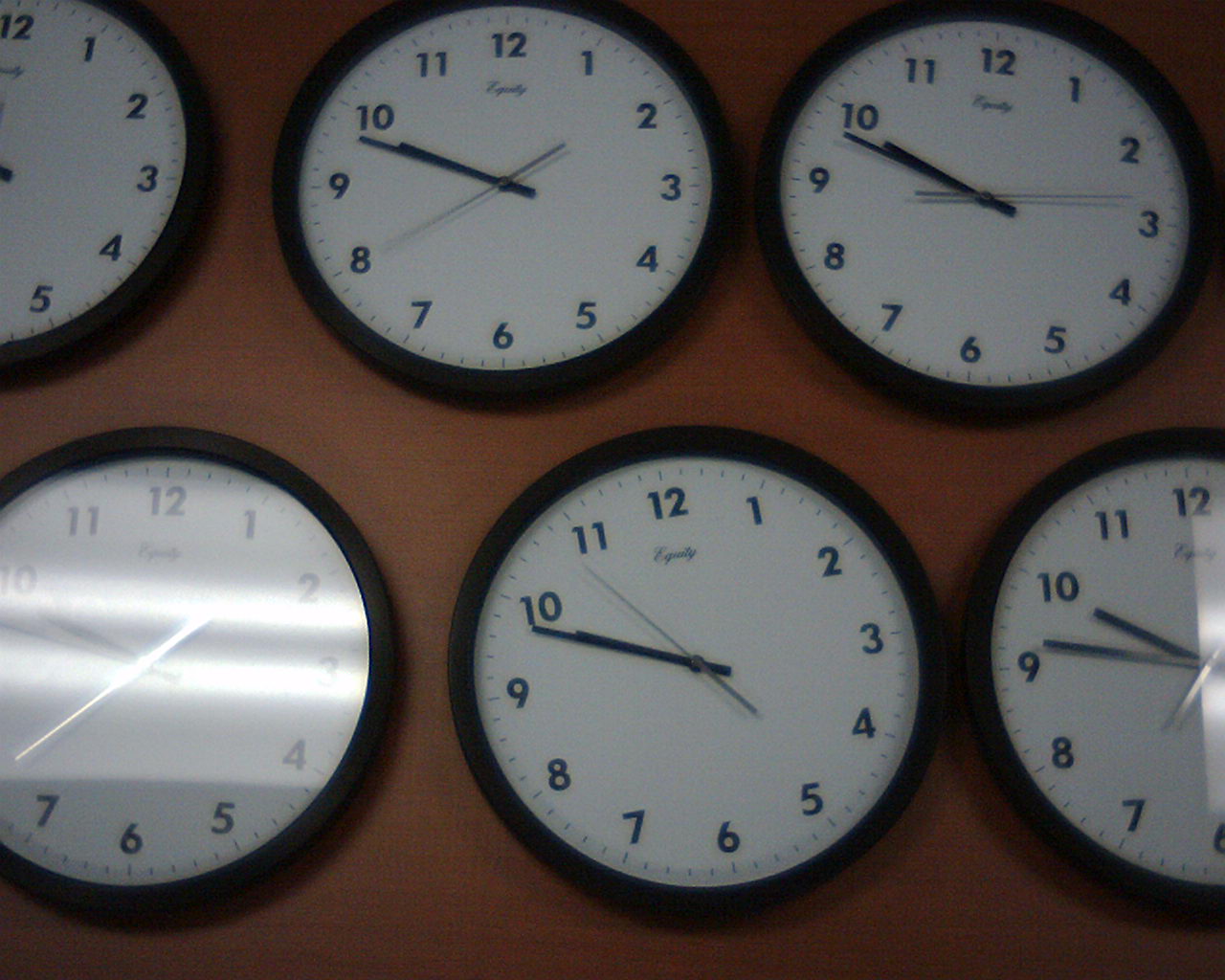This is a detailed horizontal photo of six identical, black and white wall clocks mounted on an orange wall. These round clocks, encased in a thin black frame, prominently feature white faces with plain black Arabic numerals. Each clock displays black hour and minute hands, along with a slender black second hand. The clocks' manufacturer name appears in cursive, resembling "equity," though it's somewhat difficult to read. All the clocks show a time close to 10 minutes until 10, with variations only in the second hand positions. Notably, the top row of three clocks has one partially visible on the left edge, while the bottom row of three has one partially visible on the right edge. Reflections of rectangular fluorescent lights are evident on the glass surfaces of some clocks. One clock on the lower left and another on the right prominently display these reflections. Additionally, soft shadows cast by the clocks create depth against the light brown wall background.